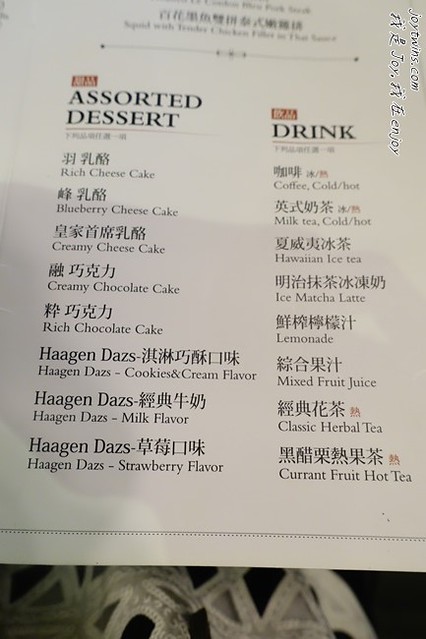The image captures a menu, prominently featuring the website "JoyTwins.com" and accompanied by Chinese characters. The menu, bordered by a delicate dotted line, rests on an indistinct surface that likely includes a patterned tablecloth. 

The menu's first column is dedicated to "Assorted Desserts," offering a variety of sweet treats:
- Rich Cheesecake
- Blueberry Cheesecake
- Creamy Cheesecake
- Creamy Chocolate Cake
- Rich Chocolate Cake
- Haagen Dazs Cookies and Cream Flavor
- Haagen Dazs Milk Flavor
- Haagen Dazs Strawberry Flavor

The second column lists an array of beverages under "Drinks":
- Coffee (Cold or Hot)
- Milk Tea (Cold or Hot)
- Hawaiian Iced Tea
- Iced Matcha Latte
- Lemonade
- Mixed Fruit Juice
- Classic Herbal Tea
- Current Fruit Hot Tea